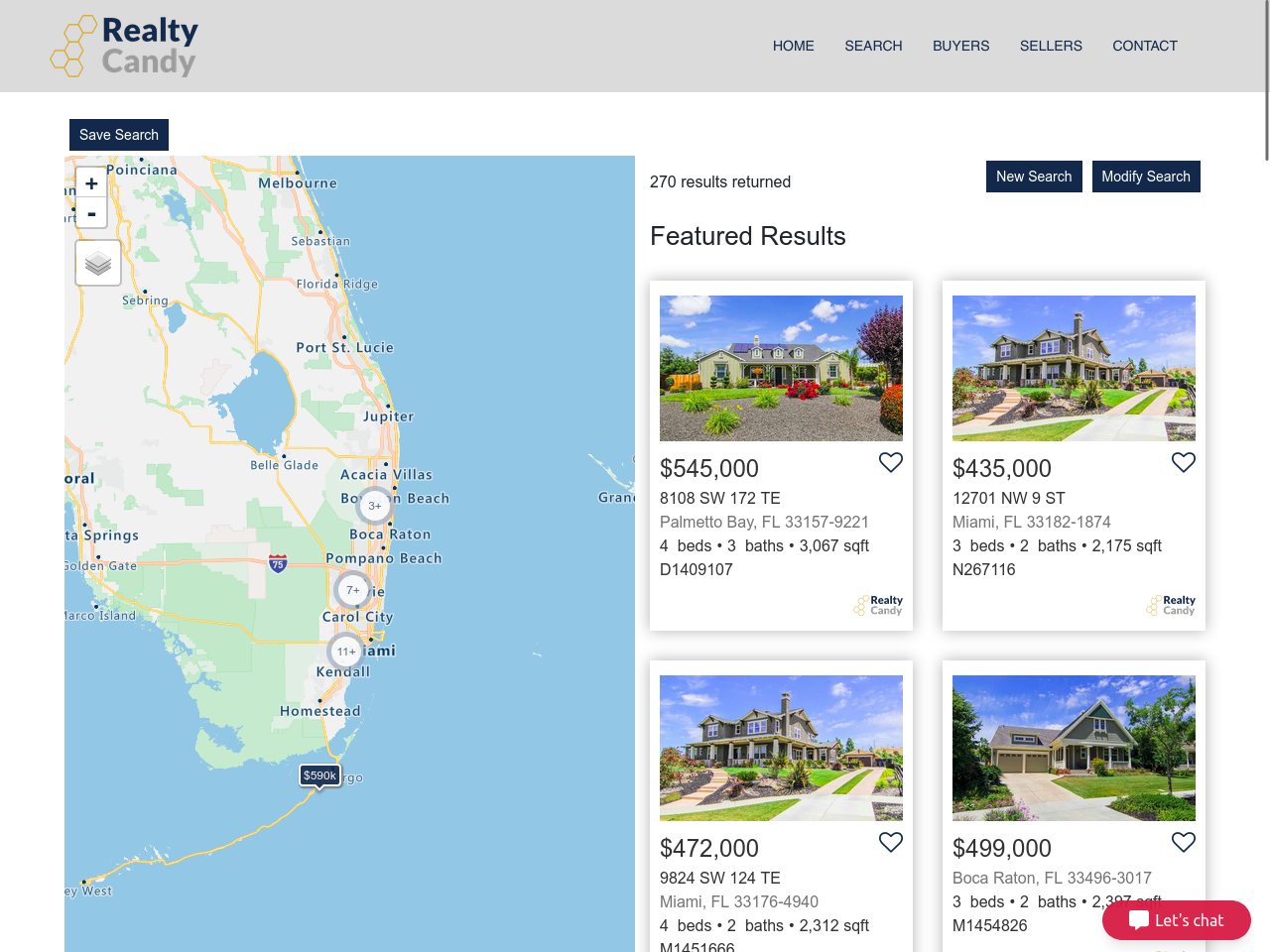**Detailed Caption:**

A screenshot from a real estate website named "Reality Candy" features an interface filled with property listings far beyond affordable reach. The website has a bluish-gray color scheme with a green DNA strand logo on the left. To the right of the logo, the site name is displayed: "Reality" in dark blue and "Candy" underneath it in a lighter hue. A navigation bar with links for "Home," "Search," "Buyers," "Sellers," and "Contact" is positioned on the upper right of the screen, containing a small vertical gray bar.

The background is predominantly white, making the text stand out. There’s a "Save Search" button shown in white on a dark blue background. Dominating the middle of the page, a large Google Map displays a section of the coast of Florida, complete with its characteristic land formations. Properties are marked on the map with gray circles featuring interior blue pop-ups showing numbers like "+3," "+7," and "+11," indicating clustered listings. A notable listing shows a price of "$590K" in a blue box with white text, situated around an island area.

On the right side, the interface indicates that "270 results" have been returned from the search. Below this, there are two blue buttons with white text labeled "New Search" and "Modify." In black text, the section titled "Featured Results" showcases four properties priced at $545,000, $435,000, $272,000, and $499,000 respectively. Each property appears grandiose, with more square footage than one could feasibly use, illustrating the tantalizing yet unattainable nature of these listings.